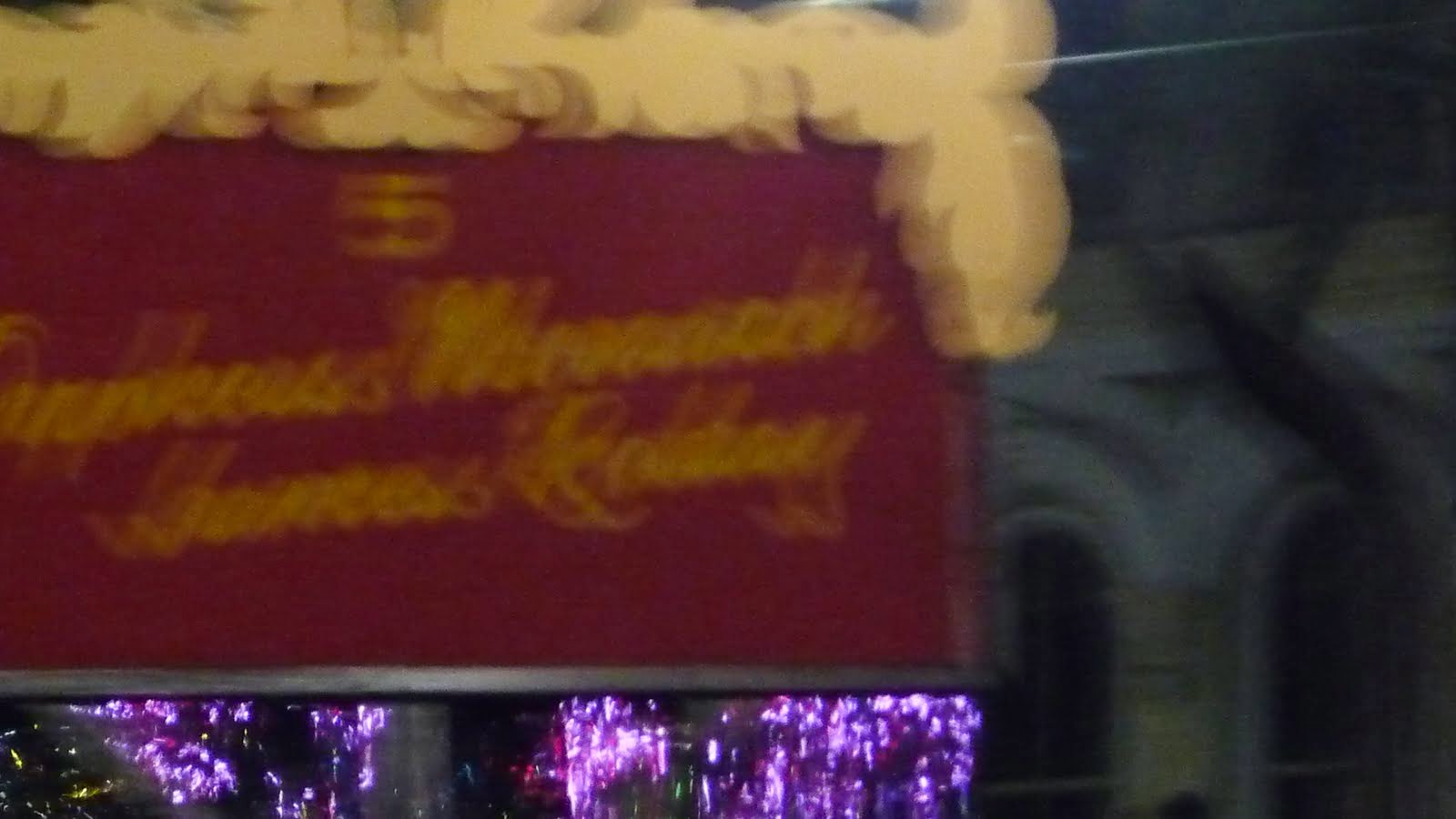This rectangular, landscape-oriented photograph is a blurry close-up of a sign positioned outside a building. The sign itself is rectangular, featuring a burgundy background adorned with yellow text. At the top of the sign, there's an ornate white decorative element attached. Below this, multiple purple lights are visible, adding a vivid, glowing effect. On the right side of the frame, part of a white building can be seen, characterized by its distinct oval-shaped windows.